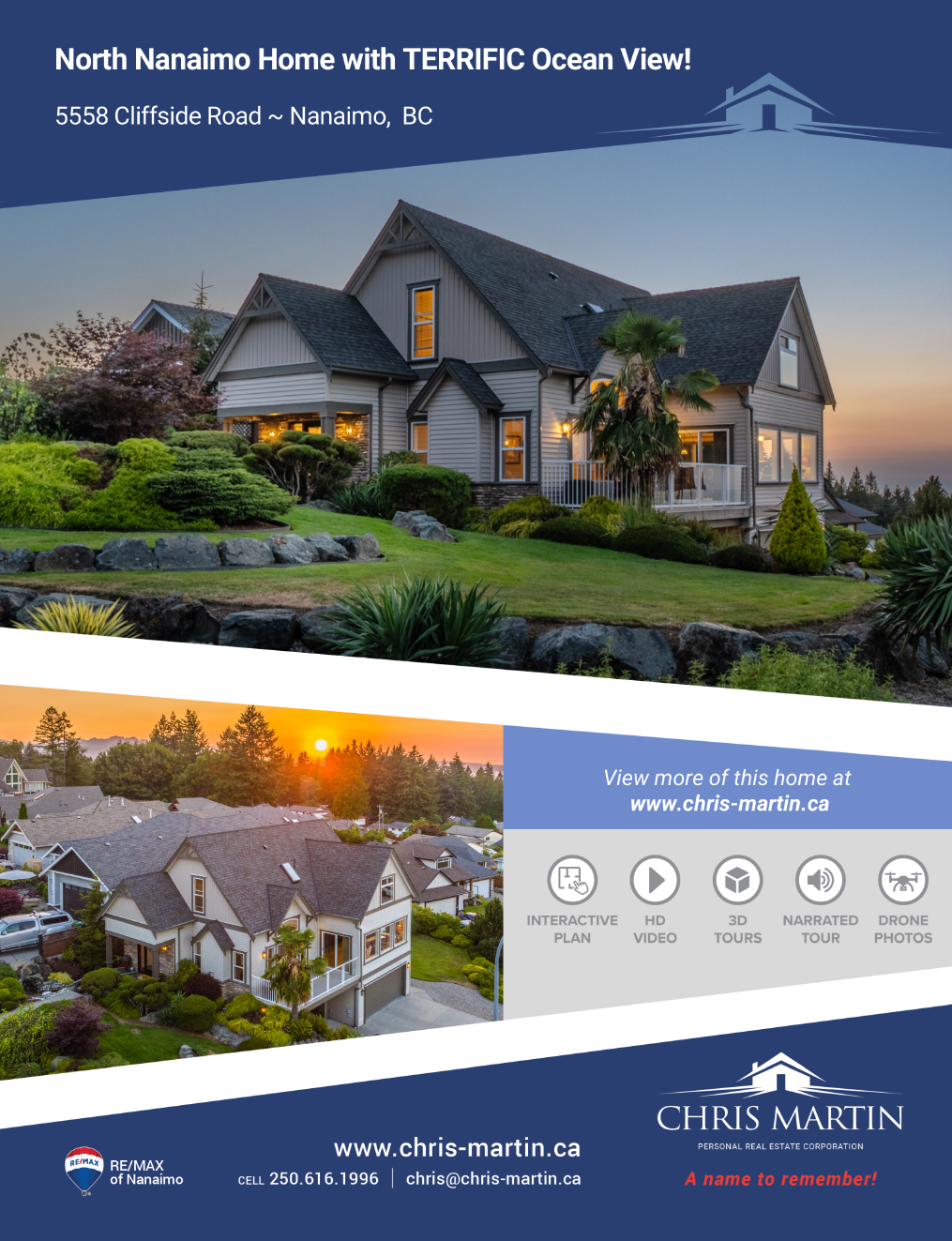This detailed advertisement for a North Nanaimo home, located at 5558 Cliffside Road, Nanaimo, British Columbia, showcases a stunning ocean view at dusk. The prominently displayed tagline "North Nanaimo Home with TERRIFIC Ocean View!" captures attention in white letters on a blue background. The house, gray with a darker gray roof, is warmly illuminated, emphasizing its inviting atmosphere. The well-manicured yard features layered landscaping with stonework and lush bushes, while the sunset or sunrise casts a pinky-orange hue across the scene. 

Below, an aerial photo offers a broader perspective of the home within its community, highlighting adjacent homes against the backdrop of a vibrant sunset. This section invites viewers to explore more through interactive floor plans, HD video, 3D tours, narrated tours, and additional drone photos available on the website www.chris-martin.ca.

In the bottom right corner, the ad features realtor Chris Martin's logo along with his contact info: cell phone and email at Chris@Chris-Martin.ca. The tagline "A Name to Remember" stands out in red, reinforcing the trust and recognition associated with the Remax brand.